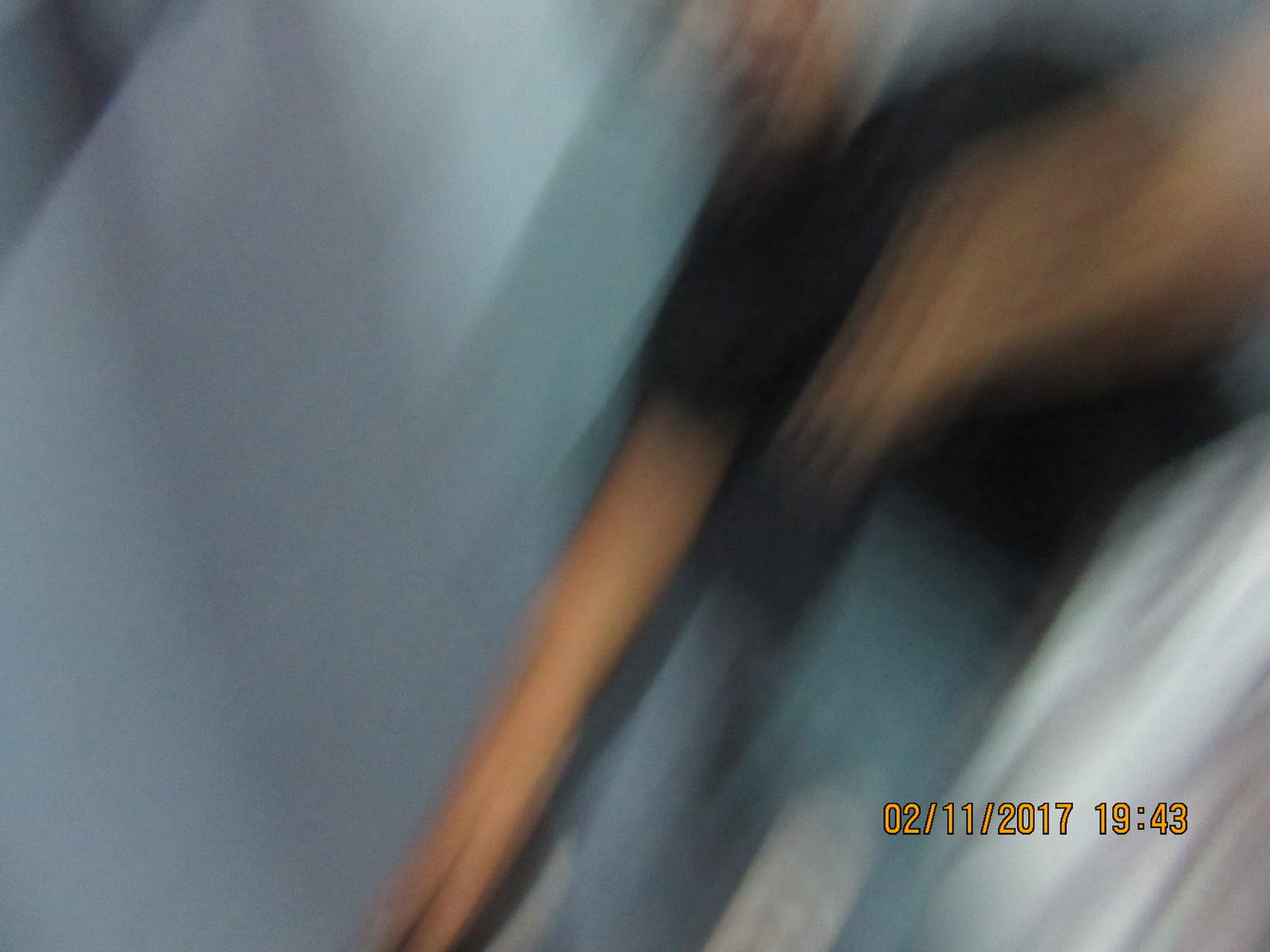This color photograph is extremely blurry and grainy, almost resembling an abstract painting. It appears to be slightly rotated at approximately a 60-degree angle to the left, making it challenging to distinguish the subjects clearly. The most visible element is a date and timestamp in the bottom right corner, overlaid in yellow ink, reading "02/11/2017, 19:43," suggesting the photo was taken on either 2nd November 2017 or 11th February 2017 at 7:43 PM.

The left side of the photograph displays various shades of bluish-grey, possibly indicating a wall or background. Towards the right, there is a vague, blurred outline of a person. This person, who appears to be male and young, is wearing a black or possibly brown t-shirt. He stands facing left, looking downward, with his right arm extending all the way to the bottom edge of the picture. His left arm bends at the elbow, bringing his hand close to his chest, as if he’s either dabbing or reaching for something.

In the bottom right-hand corner, there are triangular motion shadows adding to the blurred effect. A light brown, tan-colored shape can be seen, which might be part of a dog's legs or tail, although it’s hard to discern. There are also white streaked, extremely blurry items at the front, which makes the foreground even less identifiable. Overall, the photograph is difficult to interpret due to its severe blurriness and graininess.